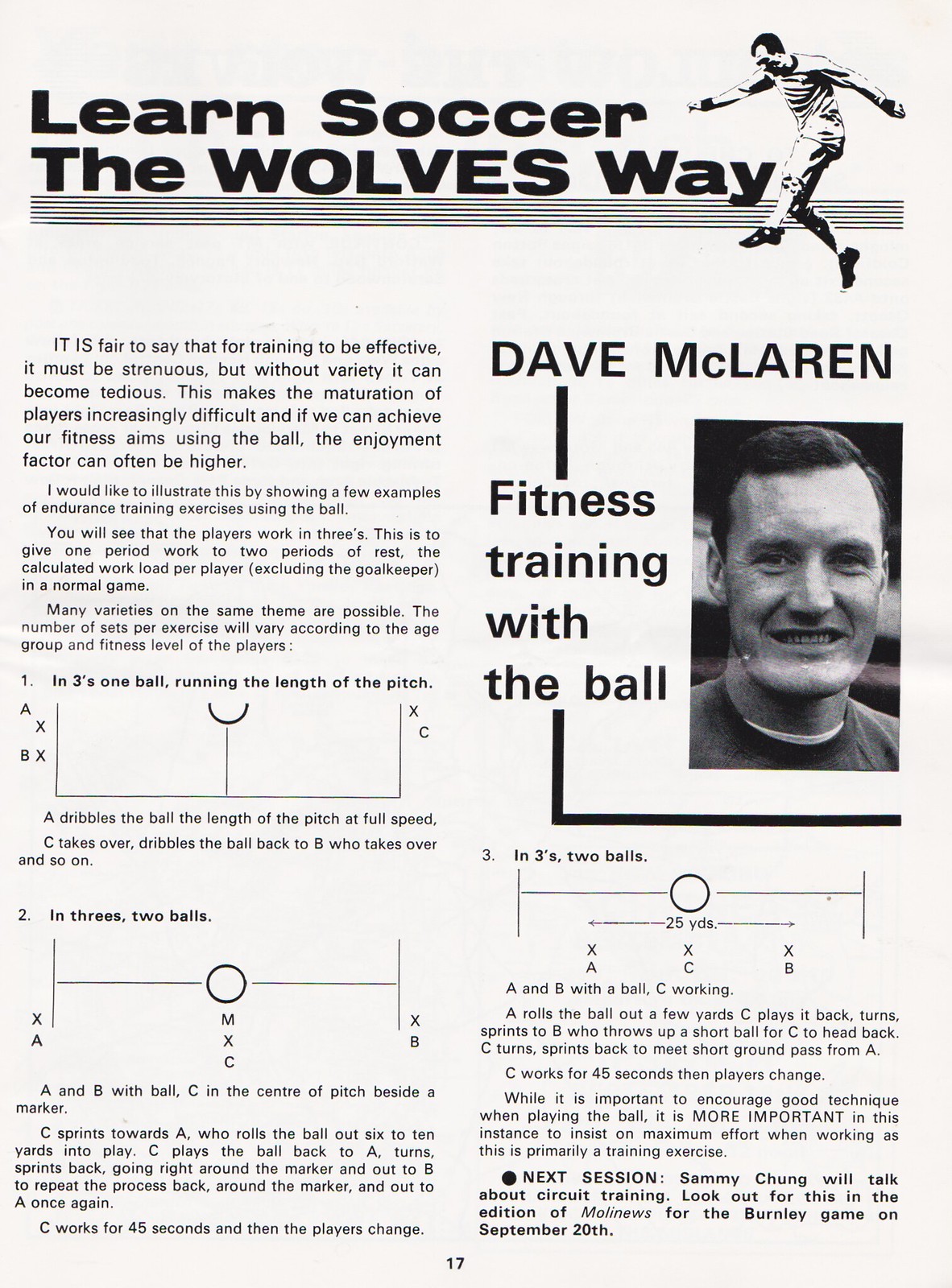This image is a black-and-white page, number 17, from a vintage soccer club program in portrait orientation. The headline, "Learn Soccer the Wolves Way," is printed in bold black lettering at the top. Adjacent to this title is a line art illustration of a soccer player kicking a ball. The page is divided into two columns of text.

In the left column, various paragraphs provide detailed instructions on soccer techniques and include two numbered gameplay diagrams labeled 1 and 2. The text emphasizes the importance of strenuous yet varied training to avoid tedium and enhance player development. It discusses how using the ball during fitness exercises can increase enjoyment and highlights the structure of these exercises, noting that players typically work in threes to allow for balanced periods of work and rest.

The right column begins with a heading, "Dave McLaren Fitness Training with the Ball," accompanied by a small black-and-white photograph of Dave McLaren—a Caucasian male with black hair, seen grinning towards the viewer. Below this photograph is another gameplay illustration, labeled number 3, followed by additional paragraphs that provide more examples of endurance training exercises, explaining how these can be varied according to age group and fitness level. At the bottom, there's a notification for the next session, indicating that Sammy Chung will discuss circuit training, which will appear in the upcoming edition of "Molly News" for the Burnley game on September 20th.